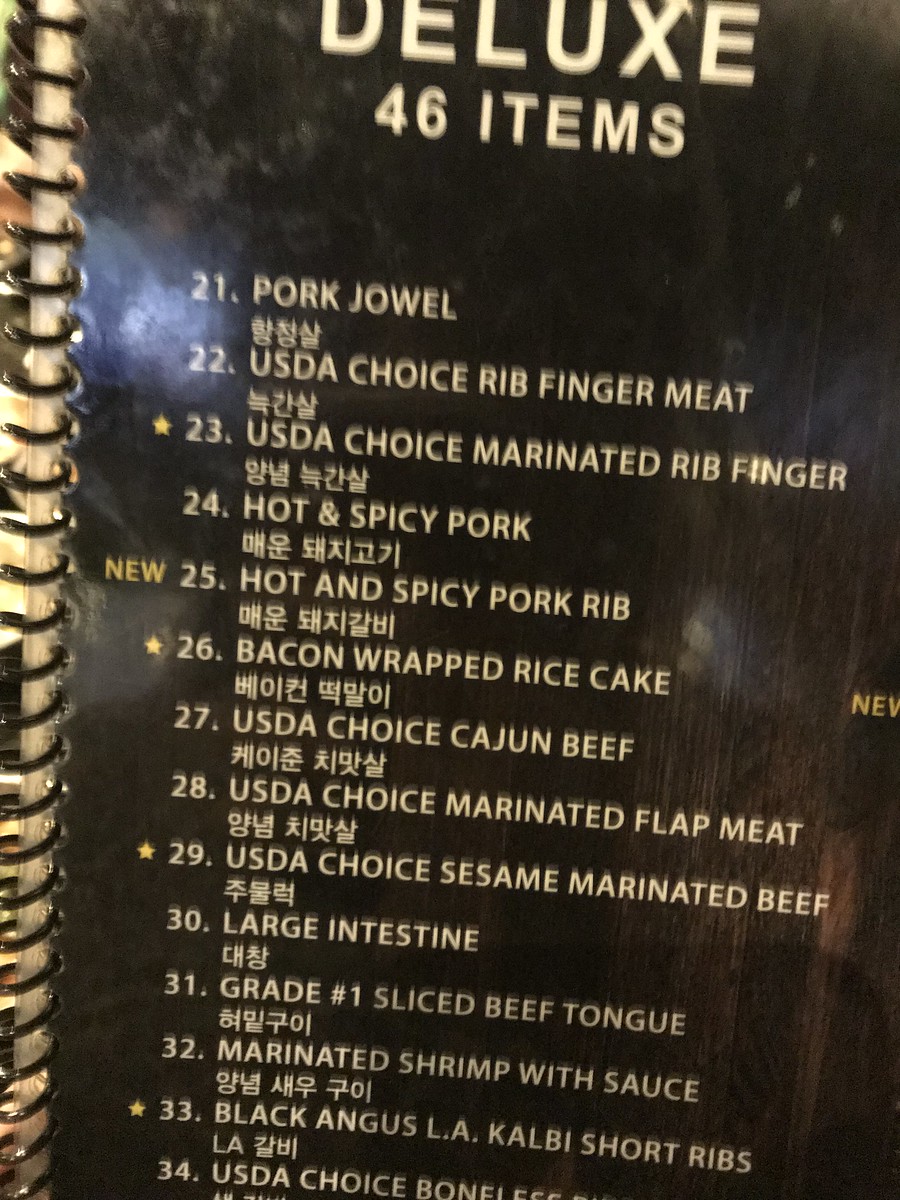The photograph captures a menu page set against a sleek, black laminated background within a spiral-bound book. Visible on the left side is the black spiral binding, and the text on the page is primarily in white bold fonts. At the top, prominently displayed, is the word "DELUXE" followed by "46 ITEMS," all written in uppercase letters. 

Beneath the heading is a list of menu items, beginning with:
- 21: Pork Chowl
- 22: USDA Choice Rib Finger Meat
- 23: USDA Choice Marinated Rib Finger, marked with a yellow star
- 24: Hot and Spicy Pork
- 25: Hot and Spicy Pork Rib, labeled as "NEW"
- 26: Bacon Wrapped Rice Cake, also marked with a yellow star
- 27: USDA Choice Cajun Beef
- 28: USDA Choice Marinated Flap Meat
- 29: USDA Choice Sesame Marinated Beef, marked with a yellow star
- 30: Large Intestine
- 31: Grade No. 1 Sliced Beef Tongue
- 32: Marinated Shrimp with Sauce
- 33: Black Angus LA Calbie Short Ribs, marked with a yellow star
- 34: USDA Choice Boneless (partially cut off at the bottom of the photo)

Each menu item is followed by writing in another language, likely providing additional details or descriptions of the dishes. The well-organized layout, clear fonts, and selective yellow stars highlight specific menu items, drawing attention to popular or recommended dishes.